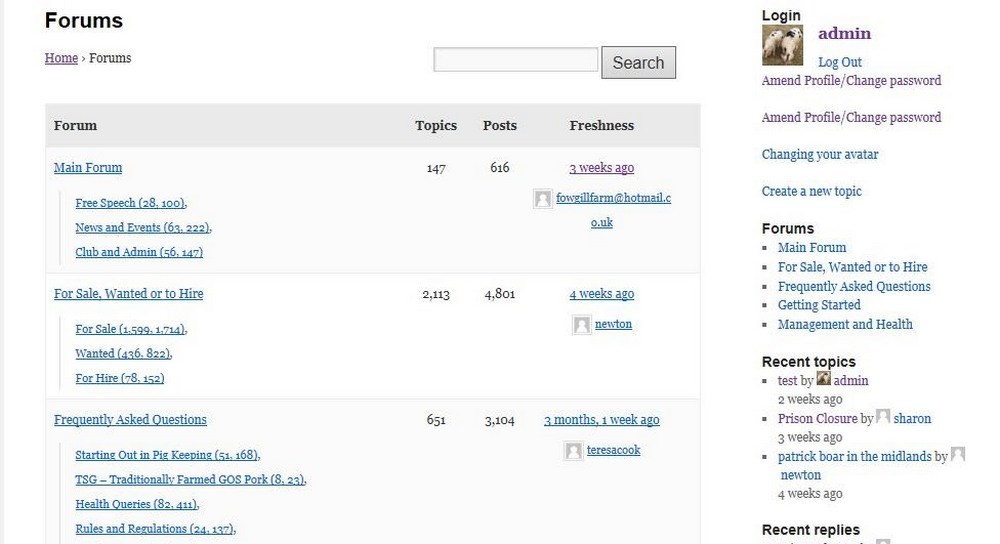This screenshot captures the main page of an online forum, meticulously divided into several well-defined sections. At the very top, a navigation bar displays the username of the currently logged-in user, reflecting their activity status on the forum.

The forum itself is structured into distinct categories, each showcasing various discussion topics. Prominently featured categories include:

1. **Main Forum:** This section comprises 147 topics and 616 posts, with the most recent activity occurring three weeks ago.
2. **For Sale, Wanted, or To Hire:** A significantly more active section, boasting 2,113 topics and 4,801 posts, with the latest interaction recorded approximately one month ago.
3. **Frequently Asked Questions:** [Details not provided in the original caption, this section would typically include numerous posts addressing common user inquiries.]

Each category is organized to display the total number of topics and posts, alongside data on the most recent activity or 'freshness' within that category. The visual layout effectively highlights the varying levels of engagement across different sections of the forum, offering users a clear overview of active and less active discussion areas.